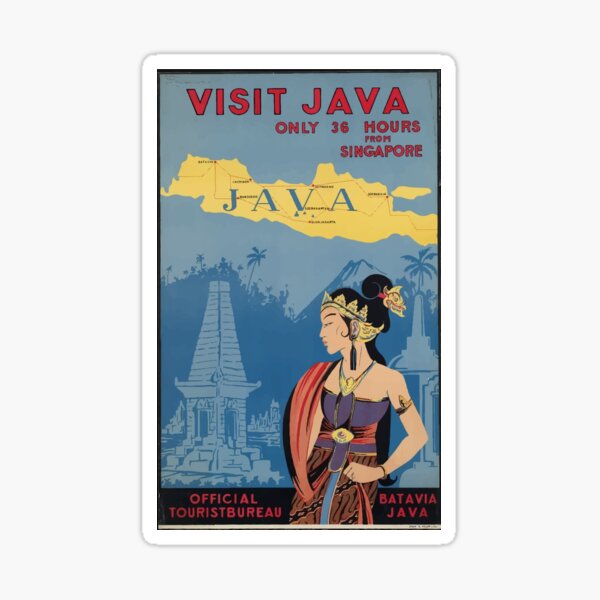This vintage travel advertisement features a central rectangular image bordered by white and black, set against a white background. At the top, in bold red letters, it states "Visit Java, only 36 hours from Singapore." Below this, the advertisement showcases a detailed map of Java in yellow, with red lines marking various locations, and the word "JAVA" prominently displayed in large blue letters.

The background of the blue poster depicts a scenic landscape with mountain peaks and palm trees, drawn in different shades of blue. On the left side of the poster, there is an illustration of a temple, and to the right, a woman with black hair is portrayed in profile. She wears an ornate gold headband or tiara, a light purple top, and a blue dress with a brass buckle. The skirt of the dress is brown, decorated with black chain designs. At the bottom of the advertisement, in red letters against a black background, are the words "Official Tourist Bureau, Batavia, Java."